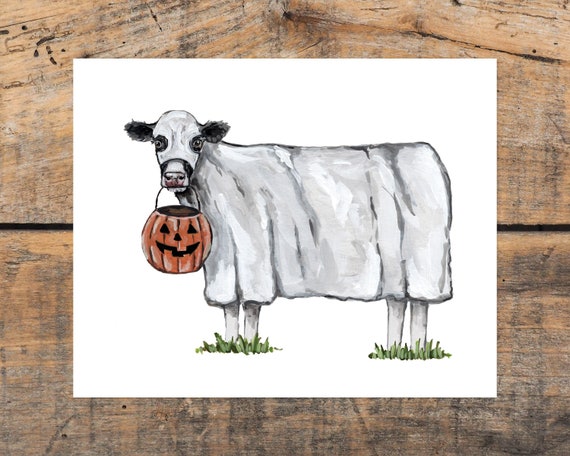This is a detailed Halloween-themed drawing of a cow on a white piece of paper, which sits on a wooden table. The cow is humorously dressed as a ghost, with a white blanket draped over its body and a white mask covering its face. Its pink nose and wide eyes are visible through cutouts in the mask, and its black ears stick out above the blanket. The cow's legs, which are white, are shown standing in patches of tall grass that reach up around them. Held in its mouth is an orange jack-o'-lantern basket, complete with missing teeth and triangle eyes and nose, emphasizing its trick-or-treating intent. The cow's head is turned to face the viewer, giving the impression that it is eagerly anticipating some Halloween treats.